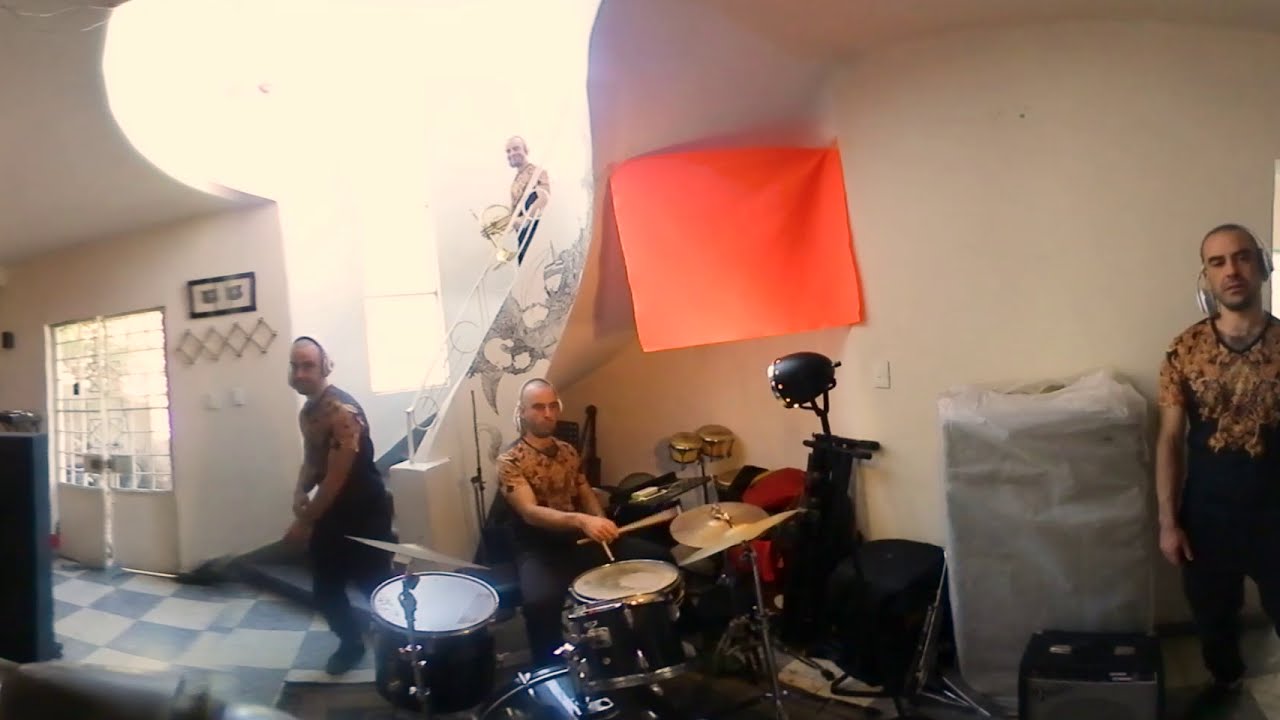In the center of the image, there's a man wearing white over-the-head headphones, a gold-colored shirt, and black pants, playing on a drum set with one drumstick on a drum and another on a cymbal. The setting appears to be inside a house with beige walls and black and white checkered tile flooring. To the left of the drummer, there is a man in a sleeveless black shirt, wearing headphones, walking towards the left and looking at the camera; he appears somewhat blurred. On the right side of the image, another man, similarly dressed in a gold and black shirt with black pants and wearing a headset, is standing against the wall and staring at the camera. In the upper middle portion of the image, there is a fourth man descending a flight of stairs, holding a French horn, although he is blurred due to the bright lighting in that area. Notably, an orange square flag hangs on the white wall behind the drummer, adding a colorful focal point to the room which is decorated with a few other items. Additionally, double doors with windows at the top can be seen on the far left, suggesting the room leads to an outdoor area.